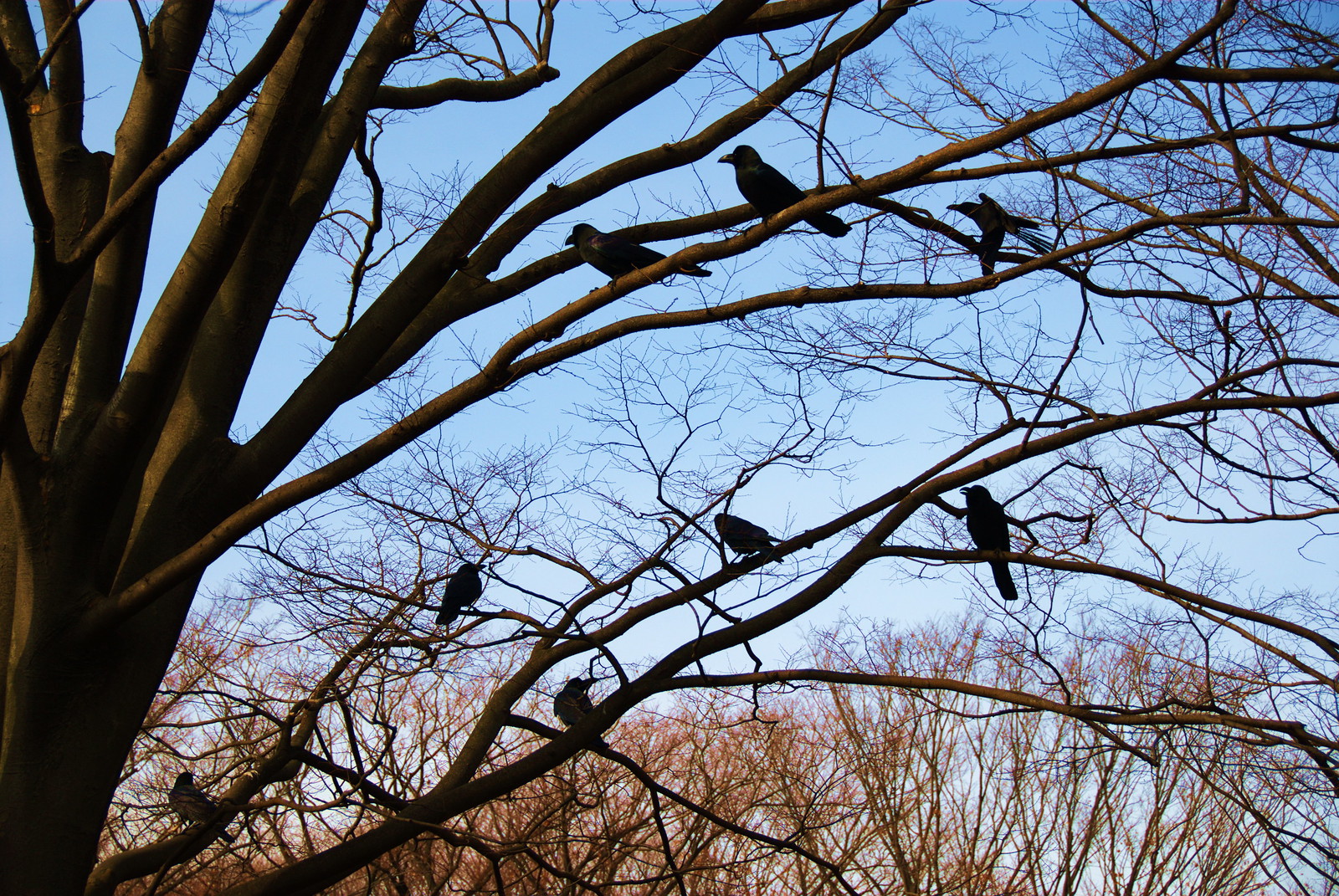The close-up image captures a canopy of leafless trees in late fall or winter, set against a light blue sky. Prominently in the foreground on the left, a large tree extends its branches upward and diagonally to the right. Among these branches, eight blackbirds, likely crows or corvids, are perched. Specifically, three birds are in the front: two share a branch, while the third flies with its wings open, head pointed to the left. Behind them, five more birds rest individually on different branches. The shot, taken slightly upward from just above ground level, also shows glimpses of other trees in the background, hinting at their sparse, brown leaves.